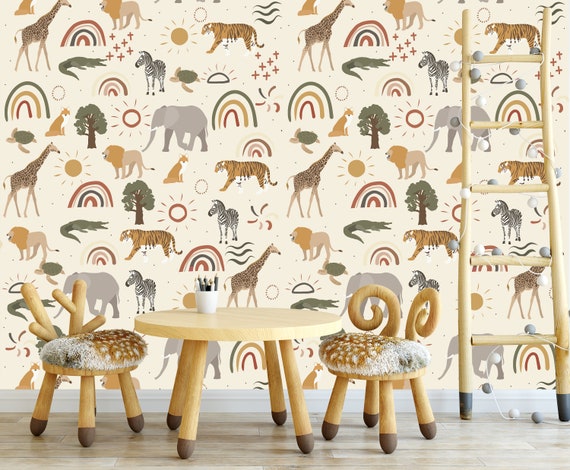The image depicts a bright, cozy children's room or playroom with a woodland theme. Dominating the background is extensive wallpaper in a warm beige or light yellow color, adorned with a rich and detailed pattern of wildlife — including dark brown and green-leaved trees, brown and black striped tigers, green alligators, black and white zebras, and brown and black giraffes in the upper left. The wallpaper also features uniquely colored elements such as green and brown rainbows, two different suns (one yellow and one red), and wavy lines that might represent snakes. 

In the center of the room, at the bottom of the image, is a charming, small, round wooden table with light brown legs that have darker brown tips resembling matches or pencils. A white container holding pens or pencils sits atop the table. Flanking the table are two adorable cushioned chairs that appear to have animal-themed designs; the one on the left has reindeer antlers, and the one on the right is reminiscent of ram horns. The chairs feature cushions with brown spotted and gray fur, evoking the appearance of fawn patterns.

To the right, there is a yellow ladder with sticks forming its sides and rungs, anchored by a black base. The room features a light brown hardwood floor with white molding at the bottom of the walls. The light in the room seems to stream from the left, casting shadows toward the right, adding to the bright and inviting ambiance.